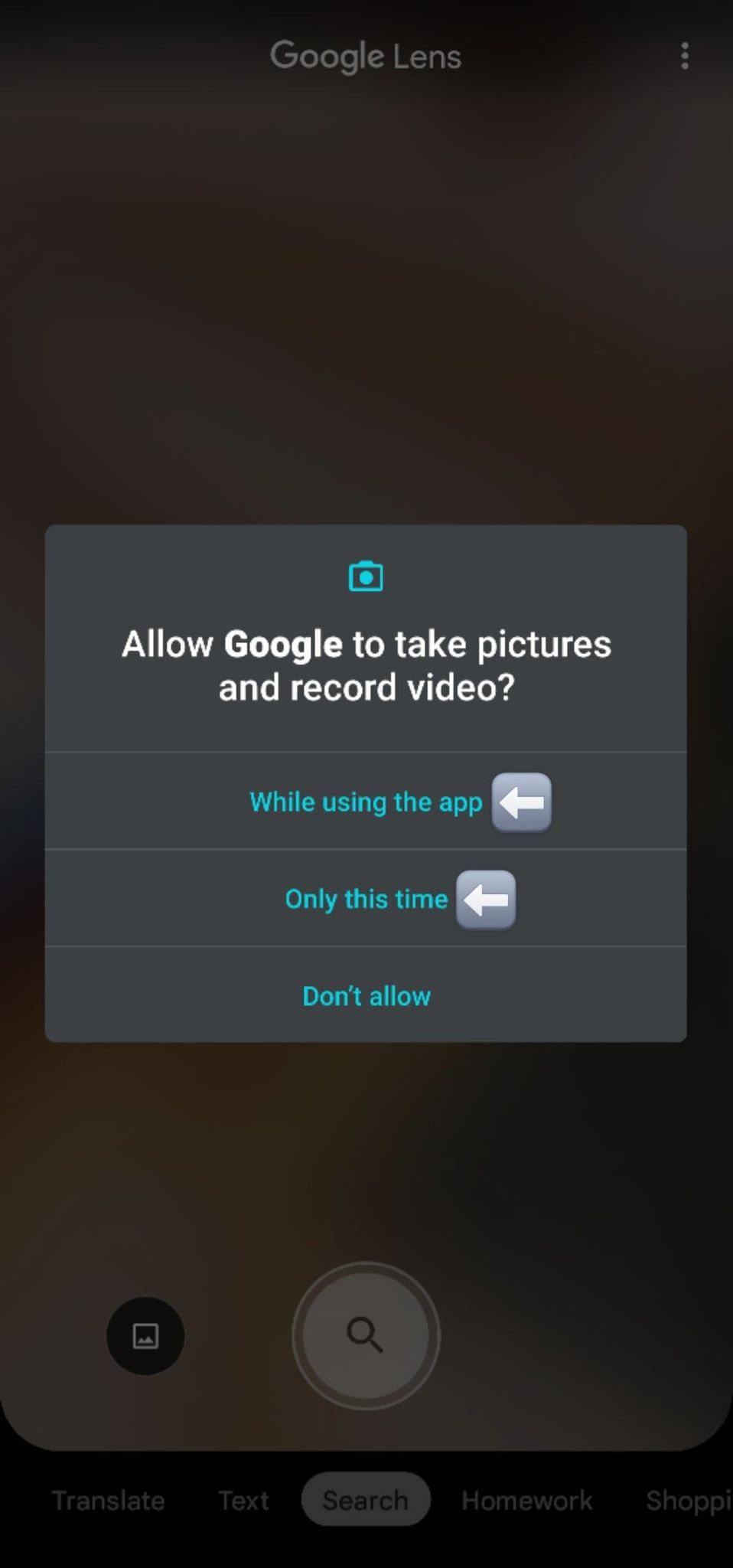This image is a screenshot from the Google Lens app, displayed on a smartphone. The background features a dark gradient that transitions from black to brownish gray. At the top of the screen, the header reads "Google Lens" in light gray text. In the upper right-hand corner, there is a vertical row of three dots, indicating a menu for additional options.

Dominating the center of the screen is a gray dialog box with a blue camera icon at its top. The text within this box prompts the user with the message: "Allow Google to take pictures and record video." Below this message are three interactive blue text options: "While using the app," "Only this time," and "Don't allow," each accompanied by a left-facing arrow symbol.

The footer of the screen contains a horizontal menu with several selectable options: "Translate," "Text," "Search," "Homework," and "Shop." Above the "Search" option, an icon resembling an hourglass inside a circle is visible, hinting at its associated functionality.